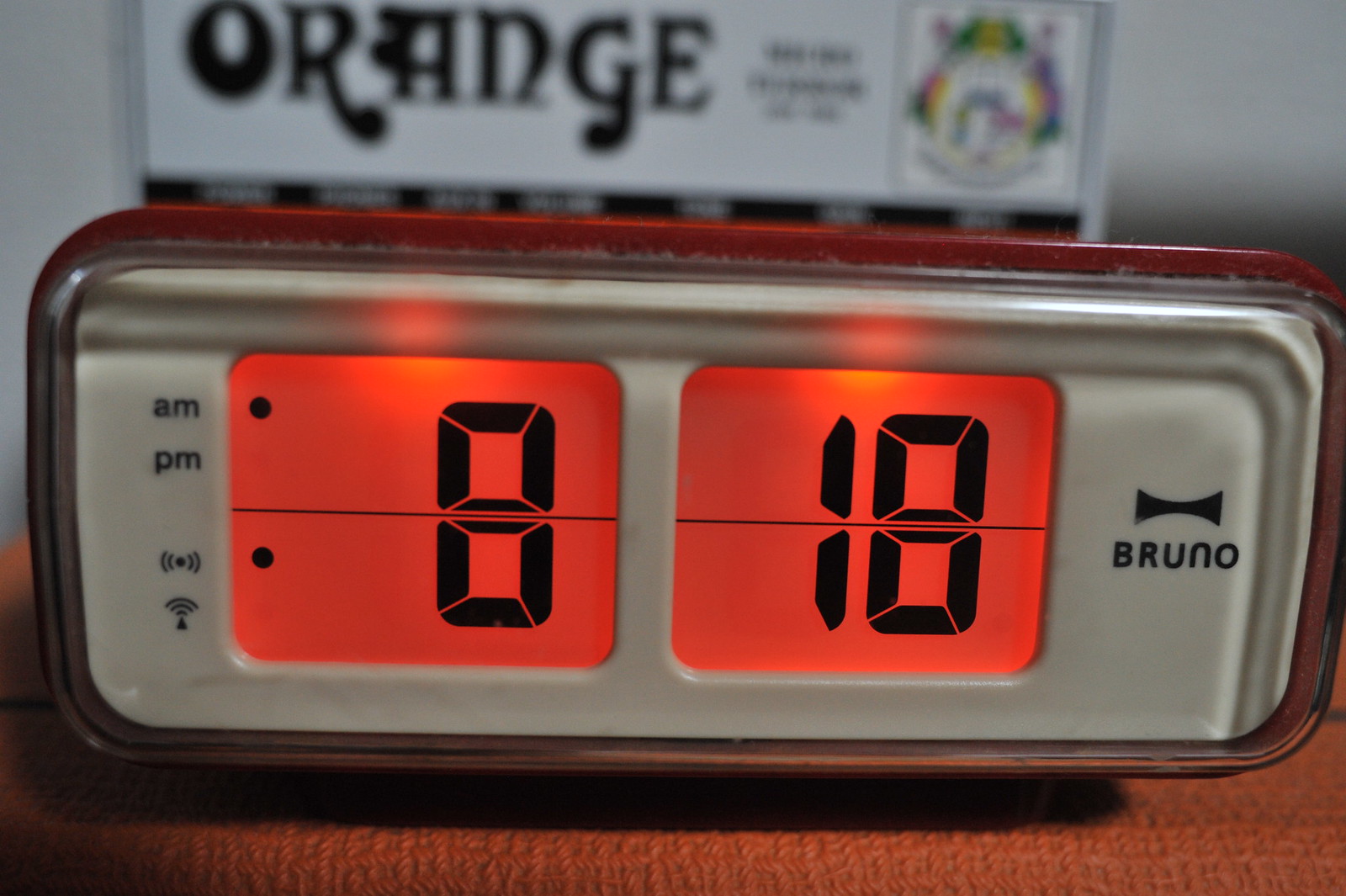Close-up of a modern digital clock with a sleek, rectangular design featuring rounded corners. The clock, positioned on a desk or table, showcases two distinct display windows separated by the clock's housing. The displays, illuminated with a soft orange background, also have rounded corners. Prominently displayed in crisp black digital numbers is the current time: 8:18. The image captures the clock's minimalist and contemporary aesthetic, highlighting its functionality and stylish design.